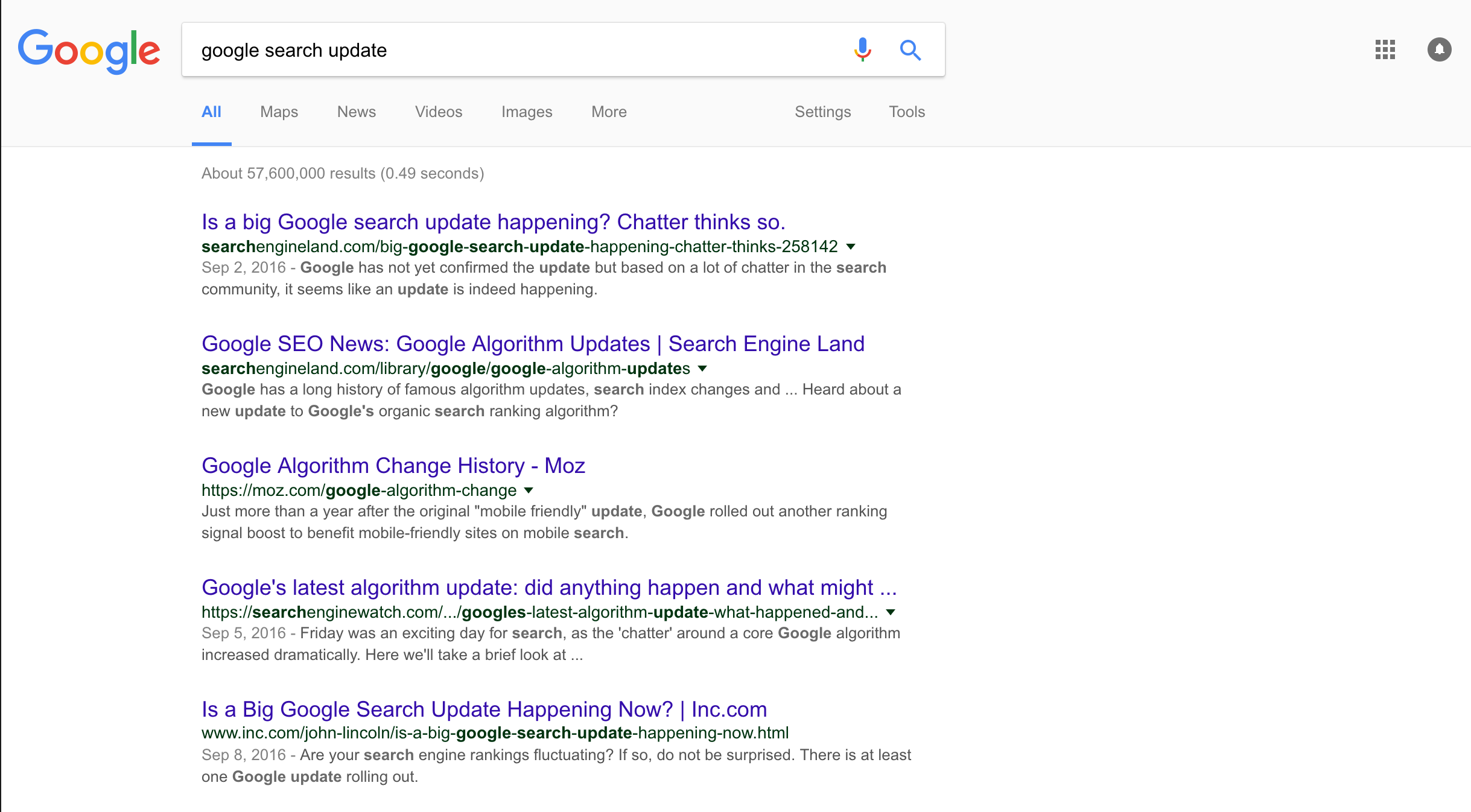The image is a screenshot of a Google search conducted on a computer or laptop, showing the search results page. In the top left corner, the multicolored Google logo is prominently displayed, followed by a search bar where the query "Google Search Update" is entered. To the search bar's right are the microphone icon and the search button, further accompanied by a grid of nine dots signifying Google Apps, and a circular profile icon.

Below this header, navigation tabs labeled "All," "Maps," "News," "Videos," "Images," "More," "Settings," and "Tools" are visible, with the "All" tab selected. The search results are listed beneath these tabs, detailing the latest updates and discussions regarding Google's search algorithms. 

The first result asks, "Is a Big Google Search Update Happening? Chatter thinks so." The second results point is "Google SEO News, Google Algorithm Updates" from Search Engine Land. The third link references "Google Algorithm Change History" from MOZ. The fourth result is titled "Google's Latest Algorithm Update: Did Anything Happen and What Might?" Lastly, the fifth result queries "Is a Big Google Search Update Happening Now?" from inc.com. Each result snippet includes brief information about the content on the respective page and indicates the date as September 2, 2016.